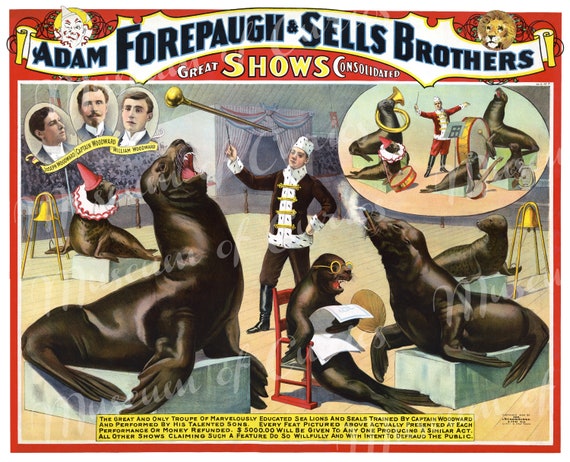This vibrant, vintage circus advertisement touts "Adam Fourpaw Sells Brothers' Great Shows, Consolidated" in bold text at the top. The scene is brimming with lively activity centered around a ringmaster in a brown conductor's uniform who orchestrates a whimsical performance by a troupe of talented seals. Four seals are featured prominently: one perches on a pedestal with a red dunce cap and white clown frills, another is mid-bark with its head raised high, and a third is seated on a red chair wearing glasses and holding a newspaper as if reading it. The fourth seal stands tall on a plinth with its mouth agape. Adding to the nostalgic charm, a detailed inset to the left showcases old-fashioned portraits of three men dressed in formal attire. The advertisement's vibrant palette of reds and yellows lends an air of excitement and grandeur, encapsulating the essence of a classic circus spectacle.